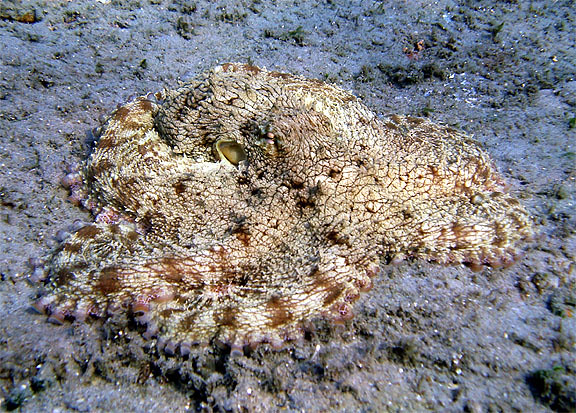A detailed and evocative description emerges from the amalgamation of perspectives: 

In this fascinating image, we observe a Caribbean octopus expertly camouflaged against the textured, blue-gray and sandy seabed. The octopus is so adeptly flattened against the surface that its elevation is barely perceptible, making it nearly indistinguishable from the surrounding environment. Its intricate texture comprises fissures, grooves, and cracks that mimic the ruggedness of the ocean floor. The creature's eye is discreetly visible, offering a clue to its presence. The coloration of the octopus ranges from creamy neutral tones to subtle browns and tans, interspersed with spots that enhance its natural camouflage. The whole scene evokes a sense of mystery, as if looking at either an underwater landscape or a surface seemingly made out of a mass of material akin to an octopus or possibly even mistaken for a shedded snake skin. The ambiguity and texture add to the enchanting and elusive nature of this marine marvel.